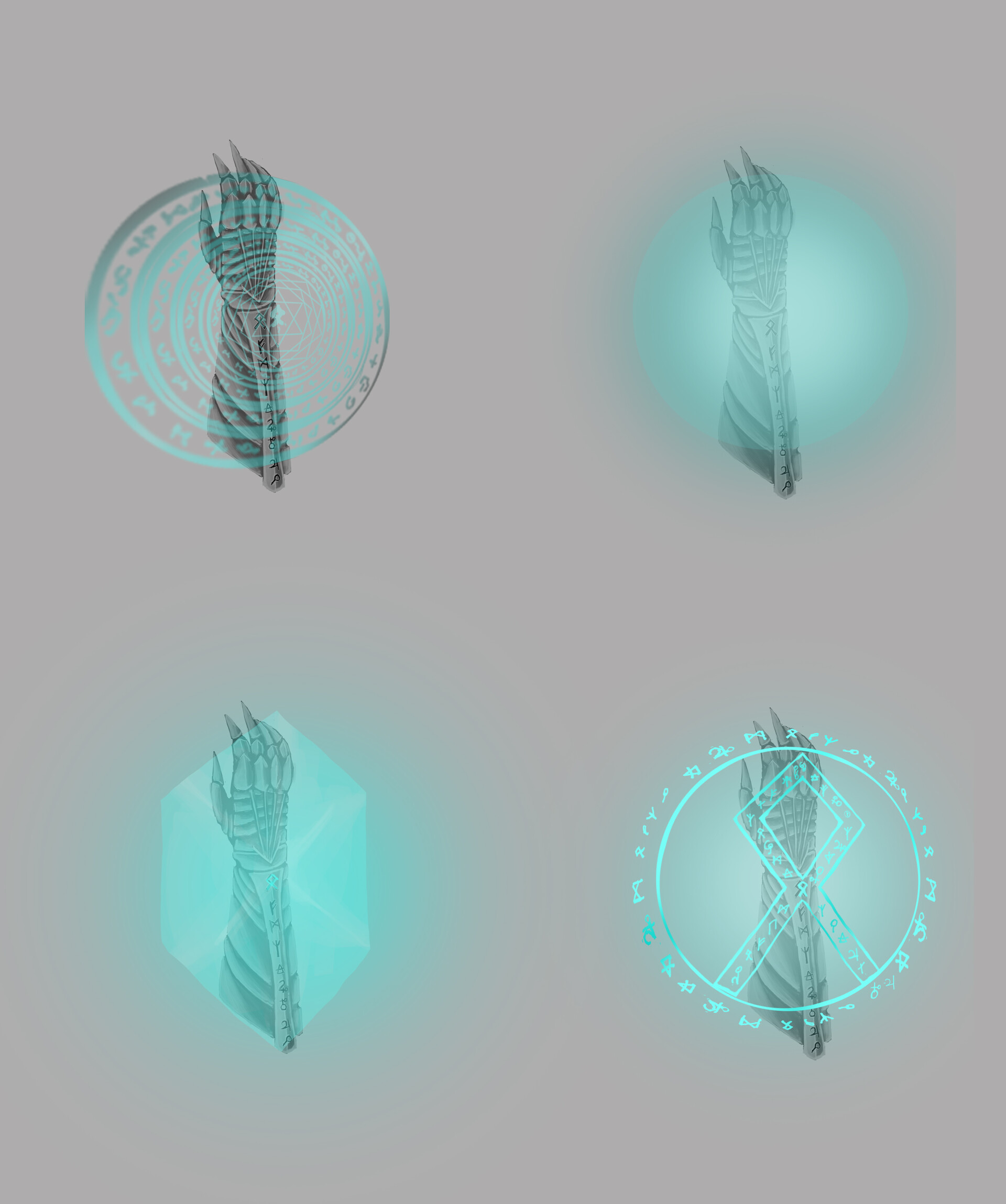This abstract composition features four reptilian-like, black hands arranged at the quadrants of a vertical, rectangular image. Each hand is cropped at the forearm and adorned with intricate, superimposed light blue and gray designs, set against a medium violet background. In the upper-left quadrant, the hand is overlaid with concentric circles containing delicate light images. The upper-right hand shares a similar circular design, featuring varying tones of light blue that create a radiant effect with a bright center and darker edges. The lower-left quadrant showcases a hexagonal light blue shape with a subtle saltire cross backdrop, adding a geometric complexity. The lower-right depicts another circular design, featuring patterns that resemble small animals surrounding a light blue knot-like figure reminiscent of an AIDS awareness ribbon. Each hand's upward-pointing fingers and detailed overlays contribute to the image's mystical and indigenous visual narrative.